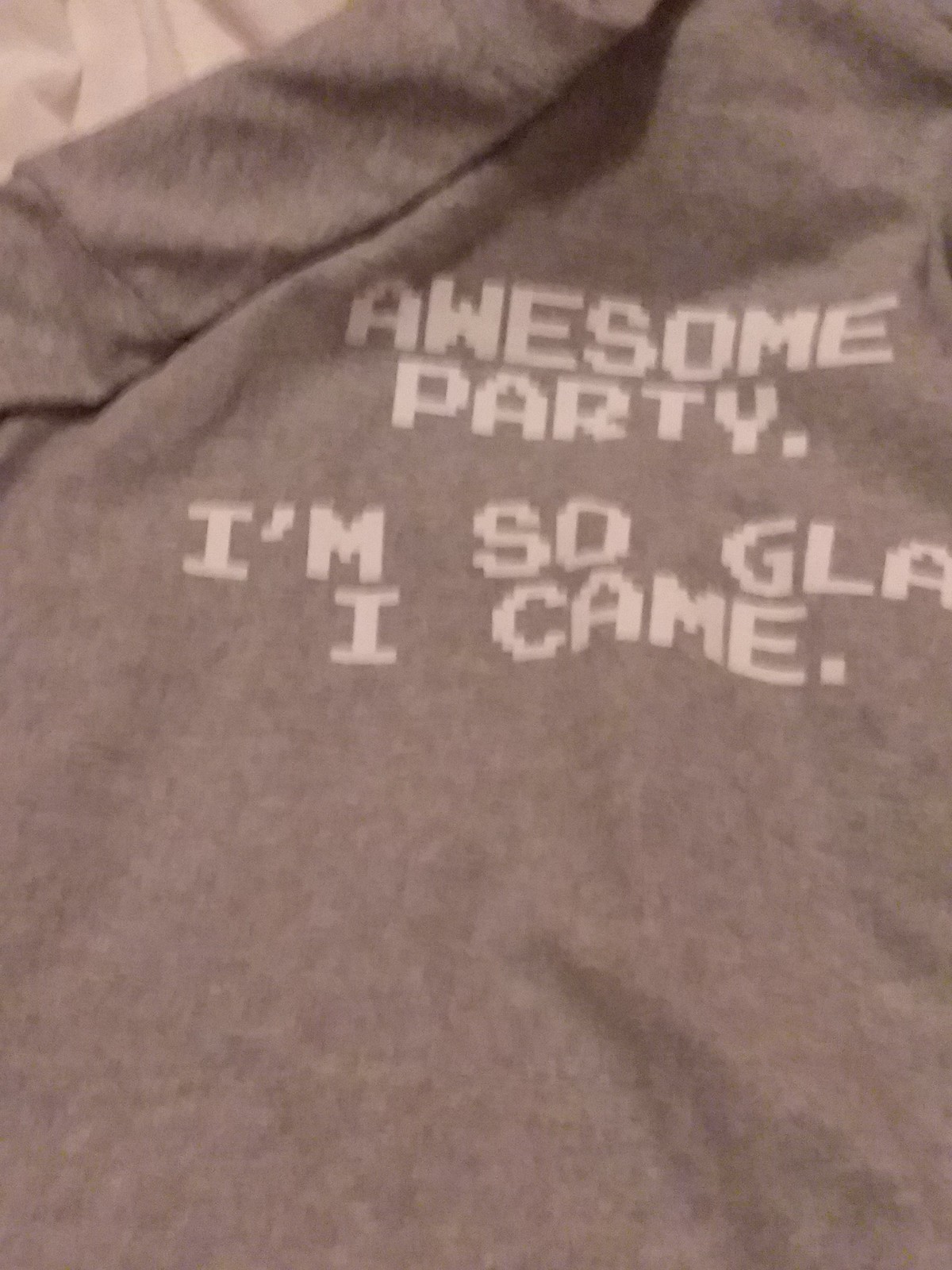This is a detailed close-up photograph of a gray t-shirt, showcasing its wrinkled and laid-out form. The t-shirt features a pixelated, block-style font that reads, "Awesome Party. I'm so glad I came." in white text. The design is printed prominently across the shoulder area, though the zoomed-in nature of the image cuts off part of the "glad" text. The shirt itself appears to be a heather gray with some lighter speckles throughout, while it sits atop a piece of white fabric that is folded in the upper left corner of the frame.